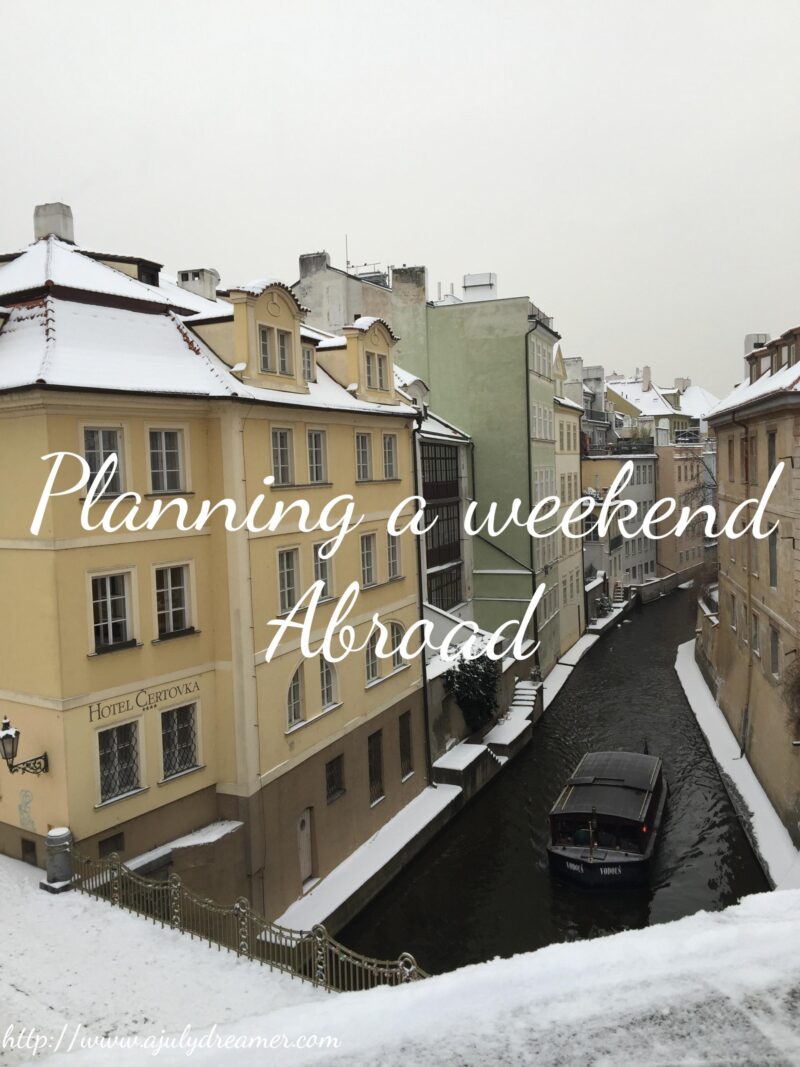In a European city blanketed in snow, a serene canal is flanked by several closely-packed, multi-storied buildings in muted hues of tan and green. A black boat, possibly a gondola, rests on the dark waters of the canal, which is bordered by buildings close enough for passengers to step out easily. Among these structures, one is distinctly marked as "Hotel Certovka" in dark brown lettering above the windows on the second story. Snow covers the rooftops, balconies, and platforms, adding to the wintry ambiance. Above this picturesque scene, the gray sky complements the tranquil setting, further enhanced by the text in white cursive that reads, "Planning a Weekend Abroad."